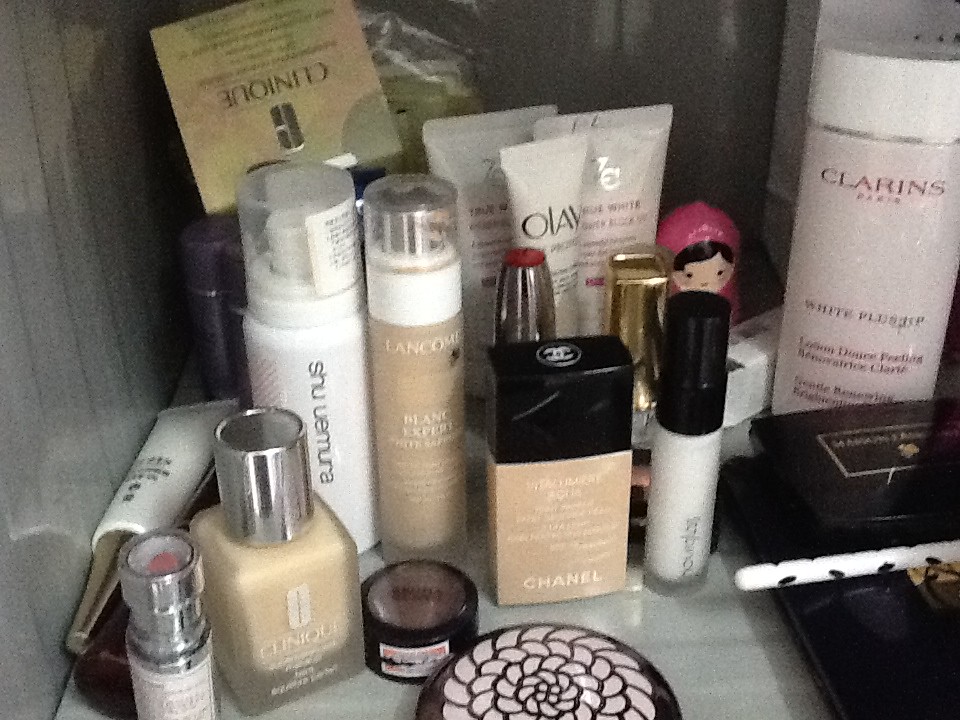The image showcases a meticulously arranged collection of makeup products displayed on an off-white table. The backdrop is a softly striped gray, positioning the setup at the table's corner. Dominating the center back is a pink nesting doll, adding a whimsical touch to the composition.

The array of beauty products spans various types, from tubes and nail polishes to concealers, representing notable brands. Prominently, Olay tubes are positioned in the middle back, accompanied by Clinique sprays and nail polishes, reinforcing the scene's high-end appeal. A Chanel foundation box takes center stage in the front, highlighting its premium status. Although most product labels are discernible, a few remain blurry and hard to distinguish.

On the right side of the arrangement, a black makeup box holds a white pencil with subtle striping. In the image's forefront lies a black compact with an intricate braided pattern and a light pink hue, adding texture to the presentation. Notably, a Clinique box and a makeup tube are tipped over on the upper and lower left, respectively, while the remaining items stand upright, maintaining an orderly appearance.

This comprehensive display of makeup products not only highlights the variety and sophistication of the items but also captures the viewer's attention through its organized yet dynamic presentation.